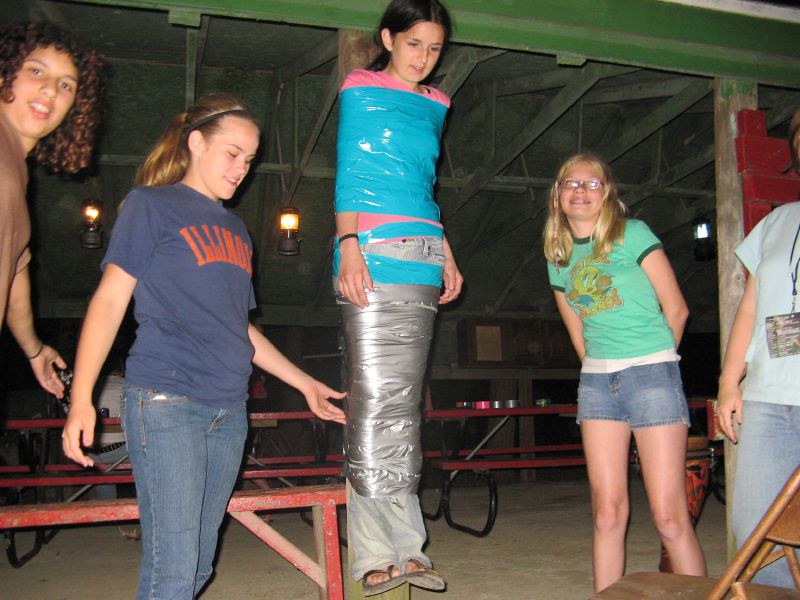The photograph shows a group of five girls, seemingly aged between 10 and 12, inside a cabin or camping building with green rafters and a wooden beam. The setting includes red picnic tables with black metal legs. One girl, wearing a pink shirt, light blue pants, a black bracelet, and sandals, is taped to a wooden beam, elevated about a foot or two off the ground. She is secured with bright blue tape around her torso and silver duct tape on her legs. To her left stands a girl barely in frame, wearing a brown shirt. Next to her is a girl in a blue "Illinois" shirt and blue jeans. On the right of the girl taped to the beam, a blonde girl in a lime green "Tweedy" shirt and blue jean shorts can be seen. The girl on the far right is mostly off-camera, visible in a light blue t-shirt and what appears to be a blue jean dress. A brown metal folding chair is in front of the two girls on the right. In the background, partially obscured, someone sits at a table in a gray shirt and blue jeans with a belt. Three lanterns hang in the back, with the left two emitting orange light and the right one either off or glowing white. The photograph appears to be taken with a flash.